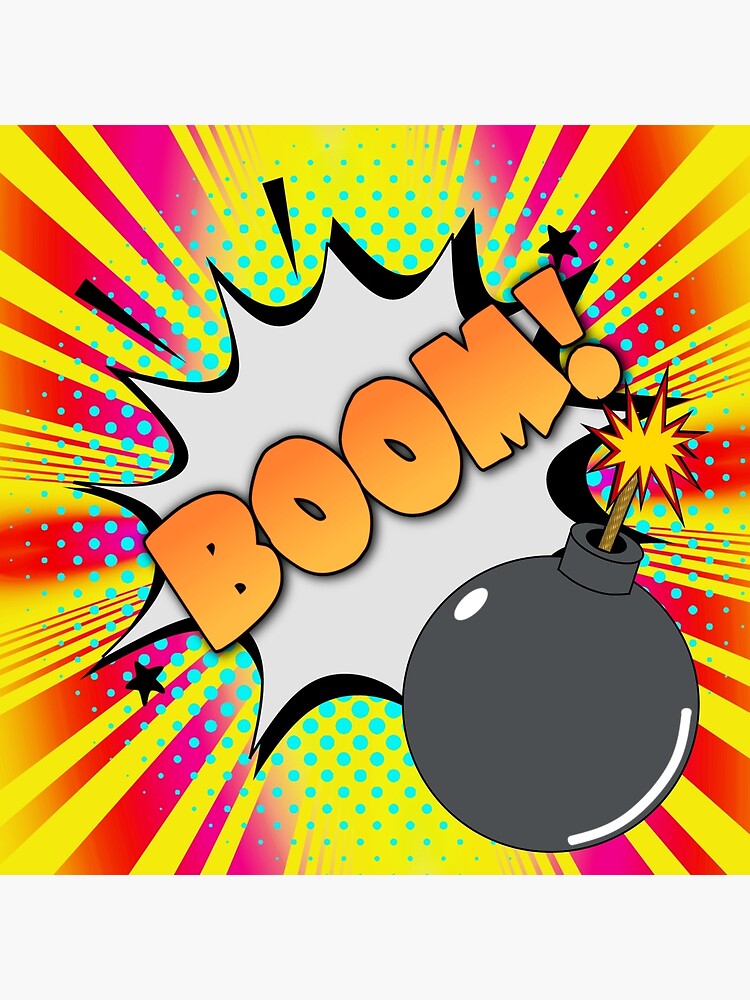In this nearly square digital illustration, a dramatic explosion scene is depicted. At the center of the image, the word "BOOM!" is prominently displayed in bold, diagonal, orange block letters. This exclamation is set within a white starburst bubble, emanating a sense of dynamic impact. Surrounding this central bubble is a dark shadow that accentuates the explosive feel. At the bottom right corner of the white area, there is an old-style bomb, colored dark gray with a burning fuse that features a yellow spark at the top, adding to the imminent sense of danger. The background vividly enhances the explosive theme with alternating rays of red and yellow spreading outward from the center. Additionally, tiny blue dots are scattered around the white starburst and throughout the image, providing an extra layer of texture and visual interest.